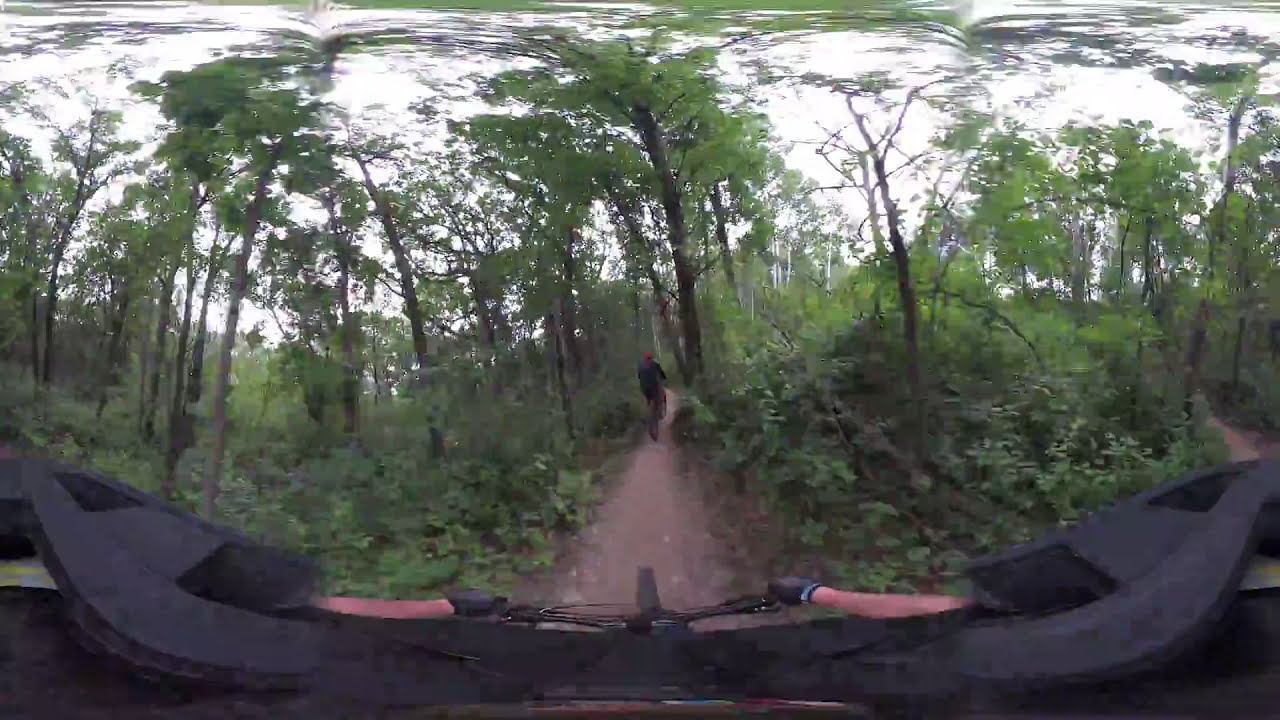This image captures a first-person view from a mountain biker wearing black gloves, navigating a narrow, light brown dirt trail through a lush forest. The perspective, taken from a helmet-mounted fisheye lens, introduces a slight distortion, curving the view at the edges while keeping the center clear. Green foliage, vines, and shrubs densely cover the ground on both sides of the path, while a mix of tall trees, some with green leaves and others bare, envelop the trail. The sky peeks through the canopy, adding a bright, white light to the scene. Ahead on the trail, another cyclist is visible, clad in a black jacket and a red cap, adding a sense of companionship to this serene yet dynamic outdoor adventure.